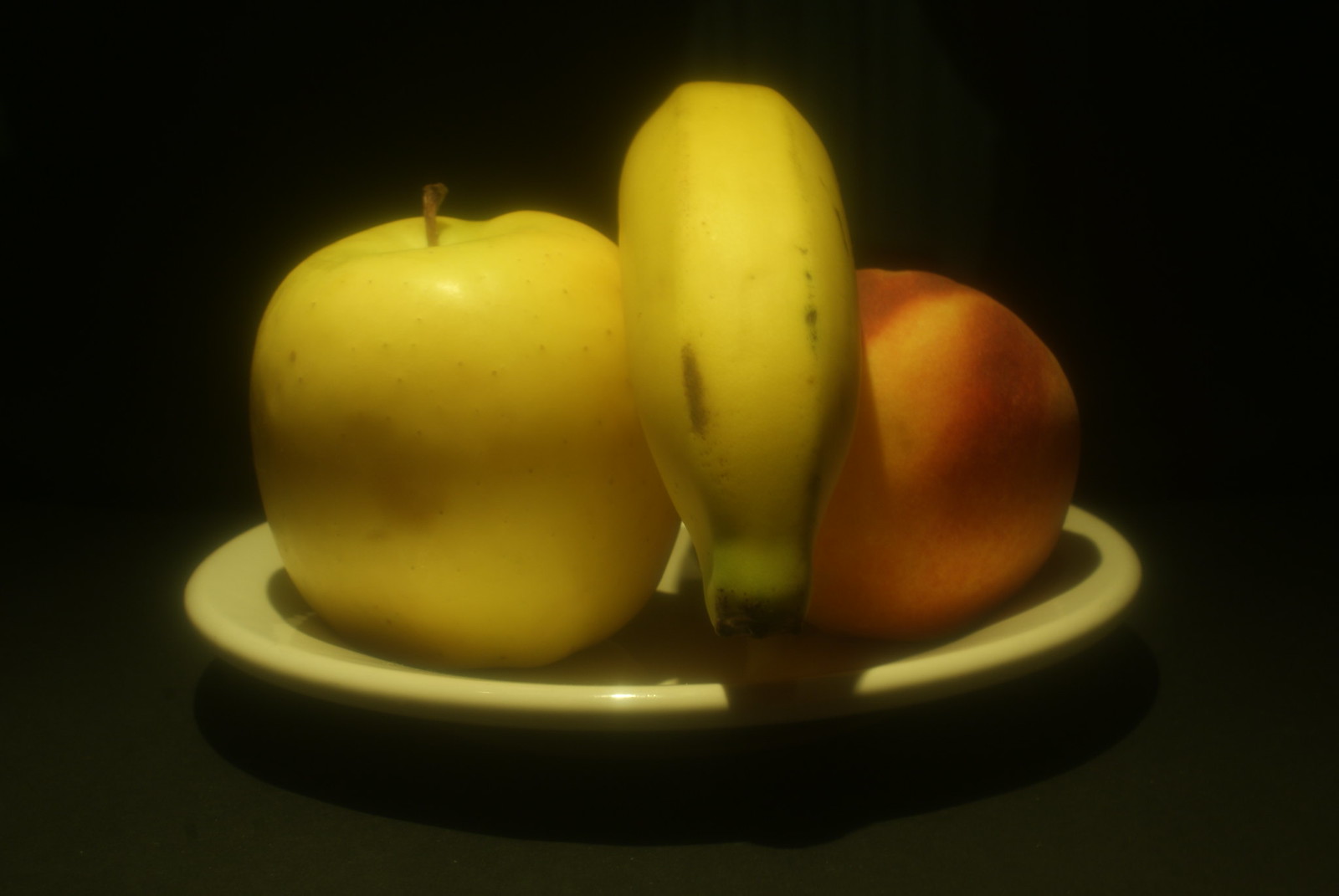In this meticulously edited studio photograph, a small white plate is showcased against a completely black background, drawing the viewer’s focus to the vibrant fruit arranged on it. From a close-up front view, we see a visually striking yellow apple on the left, a centrally positioned banana exhibiting hues of yellow with subtle green tinges, and a red and yellow peach on the right. The dark backdrop contrasts sharply with the plate and its colorful contents, making each fruit pop with a soft, glowing effect. This image has been subtly enhanced to accentuate the colors and clarity, creating a visually appealing composition that artfully highlights the natural beauty of the fruits.